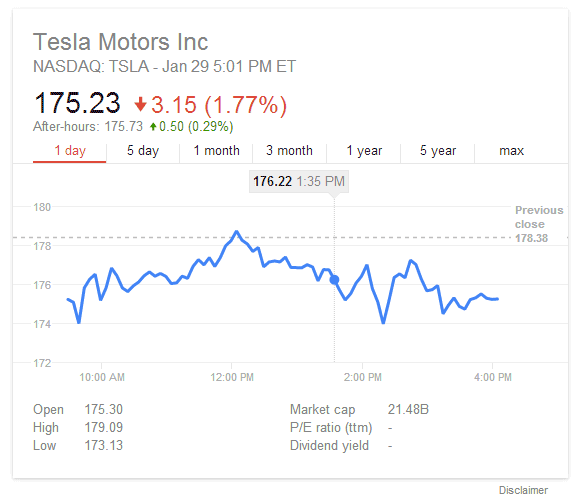This cropped desktop screenshot focuses on the financial performance of Tesla Motors Inc. (NASDAQ: TSLA) as of January 29th, captured precisely at 5:01 p.m. Eastern Time.

The main section of the screenshot displays Tesla's stock price at $175.23, highlighting a decrease of $3.15, which represents a 1.77% drop, with the negative figures shown in red for emphasis. Below this, the 'After Hours' data indicates the stock price slightly rebounded to $175.73, an increase of $0.50 or 0.29%, with these positive changes displayed in green.

At the bottom of the screenshot, there are several charting options. The '1 Day' view is currently selected and highlighted in red, while other time frames such as '5 Day,' '1 Month,' '3 Month,' '1 Year,' '5 Year,' and 'Max' are shown in black and are not selected. 

The graph below this section tracks the stock's intraday performance from 10 a.m. to 4 p.m. The chart visually illustrates a previous close of $178.38 with a blue line that fluctuates throughout the day, showing specific data points like $176.22 at 1:35 p.m.

Additionally, key stock statistics are provided:
- Opening price: $175.30
- Day's high: $179.09
- Day's low: $173.13
- Market cap: $21.48 billion
- Price-to-Earnings (P/E) ratio and dividend yield are not displayed (marked as TTM and not specified).

This detailed screenshot reflects real-time and after-hours tracking of Tesla Motors' stock performance, emphasizing daily fluctuations and key financial metrics.